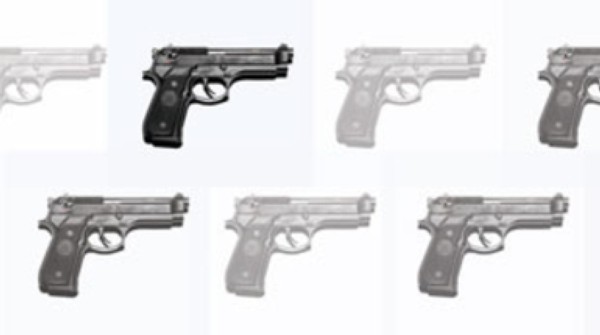The image displays a grid of seven handguns set against a white background. Arranged in two rows, the top row consists of four images where the two side images are cut off, and the bottom row features three images, forming a grid-like shape. Each handgun is a modern, short pistol with a dark handle and a metallic barrel and trigger. The guns are depicted in varying degrees of transparency and grayscale, contributing to a gradient effect. The image to the upper left is the most prominent with a dark handle and silver barrel, casting a light shadow. Nearby images show varying visibility; the ones on the edges are cut off, and the guns in the lower row also differ in shading, adding depth to the arrangement. The background sections are lightly divided, enhancing the contrast between the different saturation levels of the guns.